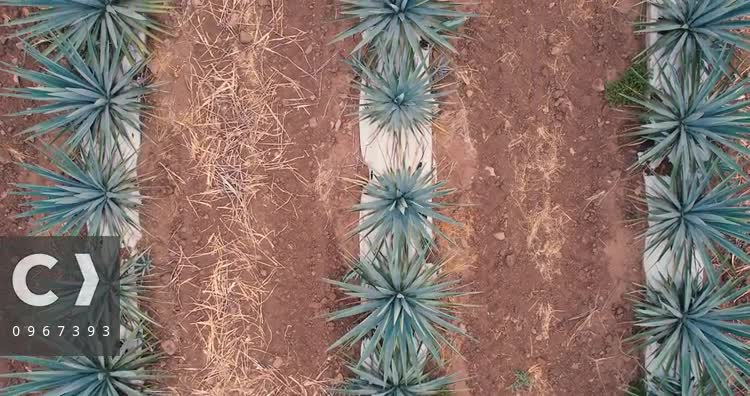The image is an aerial photograph taken outside during the daytime, capturing a deliberate, artistic setup. The landscape is predominantly a terracotta-colored clay ground, with some hay-like organic matter scattered across it. Three vertical rows of succulent plants, with an aqua green hue, are the main focus of the image. Each row is evenly spaced: one on the left, one in the middle, and one on the right. The succulents have long, thin, pointy leaves that radiate outward like starbursts. Each row of plants appears to have a white vertical strip running beneath them, though the exact nature of these strips is unclear. To the left and right of each row, there's exposed dirt; some patches contain straw, while others are bare. In the bottom left corner of the image, there is a semi-transparent gray square displaying a large white “C” followed by a right-pointing arrow and the number “0967393” beneath them.